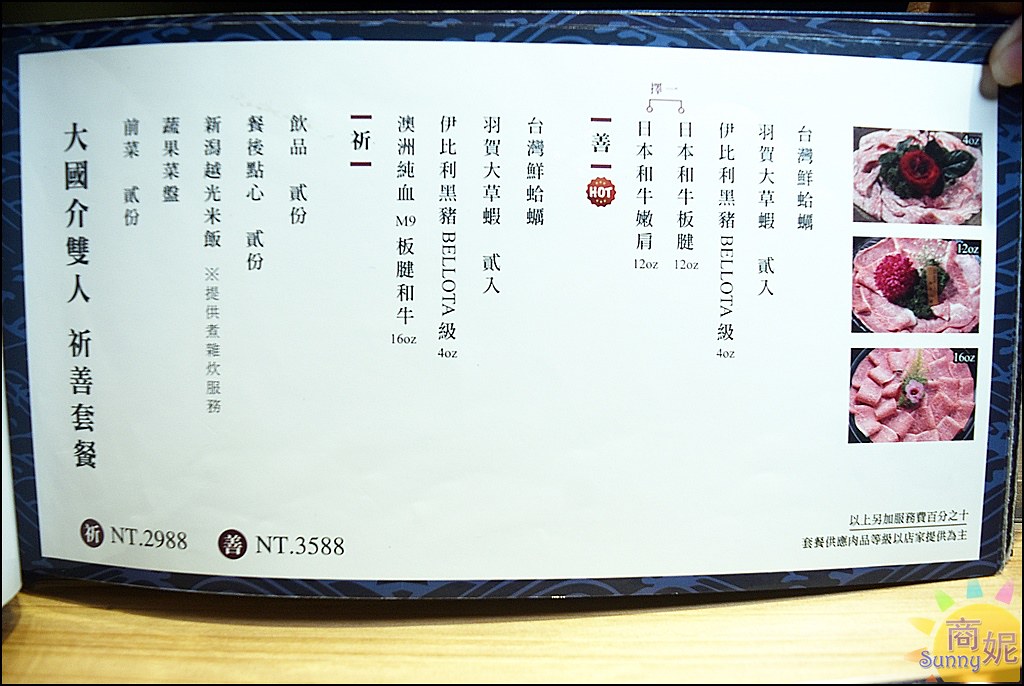The rectangular photograph depicts a menu, likely written in Chinese or Japanese, held up in the upper right-hand corner by a hand, with the thumb visible. The menu itself, placed against a light woodgrain table or shelf, features a mix of foreign characters and some English text, specifying different item weights - "M9, 16 oz.", "Balota, 4 oz.", "12 oz.", "4 oz." - suggesting it is detailing various options and sizes of food items. The notable red badge with white text marks one dish as "hot." On the right side of the menu are three images of charcuterie-like plates, displaying folded meats and labeled with their respective sizes: "4 oz." for the first, "12 oz." for the second, and "16 oz." for the third. In the bottom left corner, prices "NT.2988" and "NT.3588" are accompanied by a small circle symbol. There's also additional foreign text in the bottom right corner. The image prominently features the colors yellow, blue, light green, pink, red, and natural wood tones.